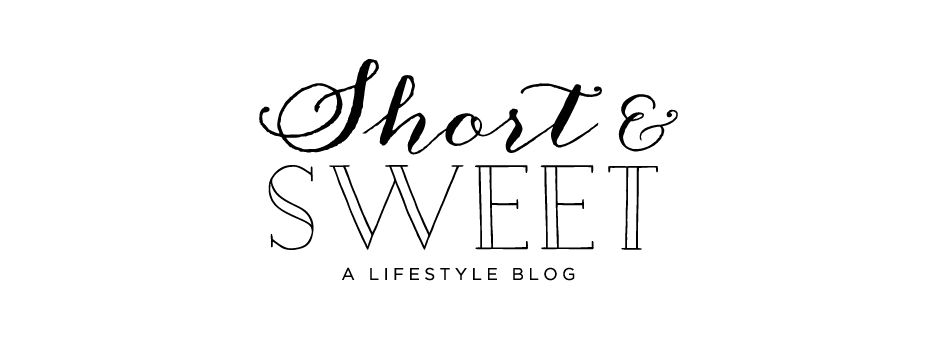This image showcases a black-and-white typography graphic design set against a completely white background in landscape orientation. The design features three centered lines of text, each distinct in style. The top line is rendered in a thick, black cursive font and reads "SHORT." Below this, the word "SWEET" is displayed in an all-caps outlined font with a slightly wider appearance. The third line, in much smaller and simpler block letters, reads "A LIFESTYLE BLOG." All text is black, with a vintage touch as the words "SWEET" and "A LIFESTYLE BLOG" appear slightly faded at the bottom left corner. The text arrangement and style suggest that this is likely a title or logo for a website or blog named "Short and Sweet."